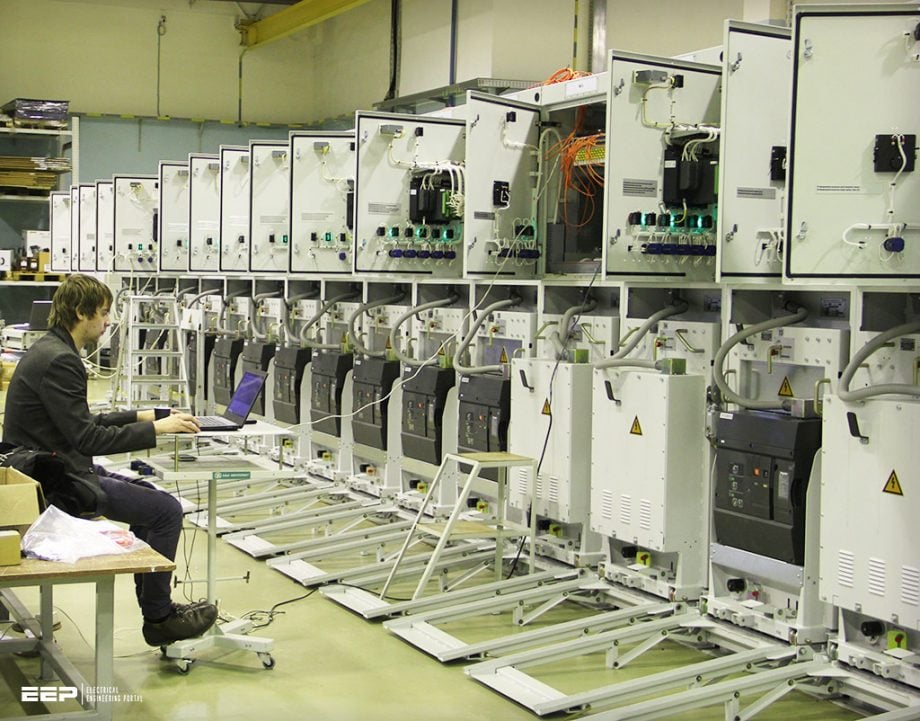The image depicts a warehouse setting with aged, yellowish walls housing numerous large appliances, likely washers and dryers, arranged in two levels on shelving units. The appliances have their doors open, revealing intricate electrical mechanisms, hoses, and circuitry, with a few doors remaining closed. A young Caucasian man with brown hair and a slight beard, dressed in dark blue or black pants, black shoes, and a black jacket or shirt, is sitting sideways on a makeshift table among boxes and plastic-wrapped items. He is intently focused on a laptop stationed on a movable workstation, connected by an electrical cord to one of the nearby machines, presumably to check connections or test the unit's functionality. The scene also features the text "EEP" in bold letters in the lower corner of the photo, accompanied by smaller, unreadable technical writing.